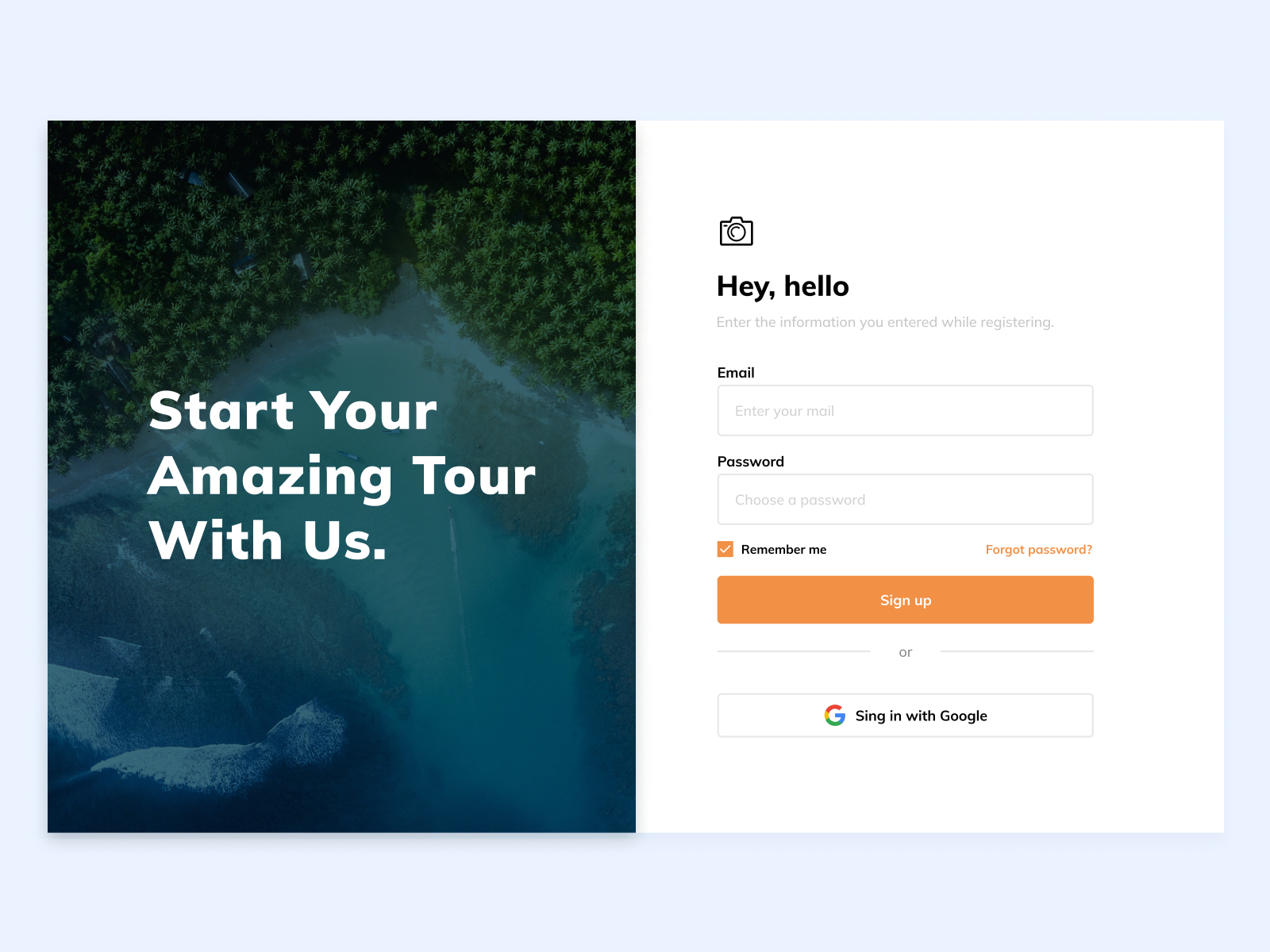This screenshot captures the landing page of a potential website or app, meticulously divided into two sections against a light blue background with subtle shadowing. The left section features a striking aerial photograph of a dense forest along a coastline, darkened to near night-time effect to enhance the centered text. The text, spanning three rows, reads: “Start your amazing tour with us.”

The contrasting right section is designed for user interaction, featuring a pristine white background populated with various elements:

1. A camera icon at the top.
2. A friendly greeting text: “Hey, hello.”
3. A subheading prompting the user to input registration information: “Enter the information you entered while registering.”
4. A form field labeled “Email” with placeholder text: “Enter your email.”
5. A form field labeled “Password” with placeholder text: “Choose a password.”
6. A checked checkbox labeled “Remember me,” situated next to a “Forgot password” link.
7. A prominent, orange “Sign Up” button with white text.
8. Divider lines and text, offering an alternative login method: “or,” followed by a slightly mistyped prompt, “Sing in with Google,” featuring the Google logo.

The design clearly differentiates the visually captivating left side from the functional, text-rich right side, guiding the user’s focus effectively through the landing page.